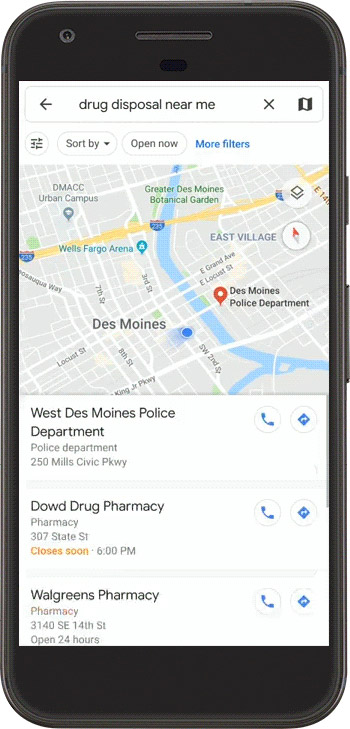The image showcases an older model cell phone with prominent black borders at the top and bottom, encased in a black bezel. The phone displays a webpage with a predominantly white background. The page features a map of Des Moines, Iowa, accompanied by a search bar at the top containing the query "drug disposal near me." Below the search bar, there are options for sorting the results, filtering by "open now," and additional filters.

The detailed map, resembling a rendered Google map, highlights various locations in Des Moines, including the Des Moines Police Department, Dow Drug Pharmacy, and Walgreens Pharmacy. The map displays the general layout of the city's streets and waterways. Beneath the map, contact options are available, including a phone icon and another unidentified icon depicted as a blue triangle with an arrow pointing to the right. Each location listed provides further details, such as addresses and hours of operation.